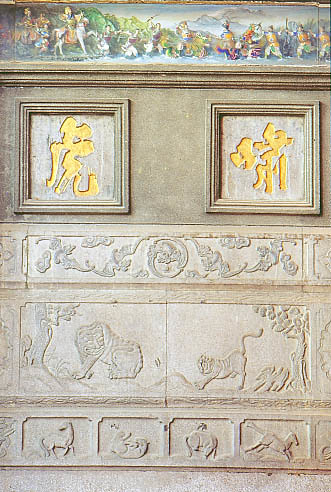The image displays a detailed, elaborate stone mural combining both painted and chiseled elements, divided into distinct segments. At the very top, a colorful rectangular panel depicts a dynamic battle scene featuring a man on a white horse charging towards a group of men running across a river, weapons raised. Below this vibrant scene, two grayish squares contain golden characters that resemble Chinese or Japanese writing, though their exact language is unclear.

Descending further, the mural transitions into a strip of intricately chiseled engravings without color, showcasing raised designs. The first engraving portrays stylized shapes resembling clouds with a central figure that could be a bird or dragon. Subsequent engravings depict pairs of animals: one area shows what appear to be two tigers, one poised to pounce while the other looks back, and another section features an elephant on the left and a leopard on the right.

At the bottom of the mural, additional engravings illustrate a series of animals, including horses that seem to change posture from looking back to rolling on their backs and eventually running away. Despite the absence of color in these lower segments, the precision and craftsmanship of the chiseled designs highlight the skills and effort invested in creating this multifaceted stone artwork.